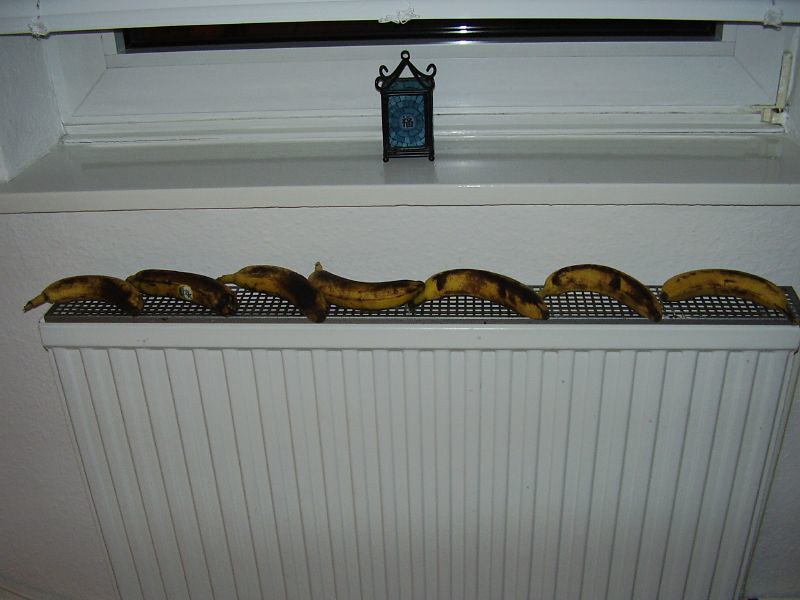This real-life photograph captures an indoor scene centered around a white recessed radiator with a silver-gray metal grate. Atop the radiator, seven overly ripe and heavily blotched bananas are meticulously lined up. The backdrop features a white stucco-textured wall beneath a window with its horizontal white blinds partially pulled down, revealing a fraction of the glass which reflects the camera's flash. Above the radiator, on a white or cream-colored marble windowsill, sits a distinctive trinket—a small, blue glass mosaic lantern with an Asian-inspired design. The lantern's rectangular sides are adorned with blue glass, and it features a pagoda-style top made of bronzed metal, adding an intriguing cultural aesthetic to the scene.